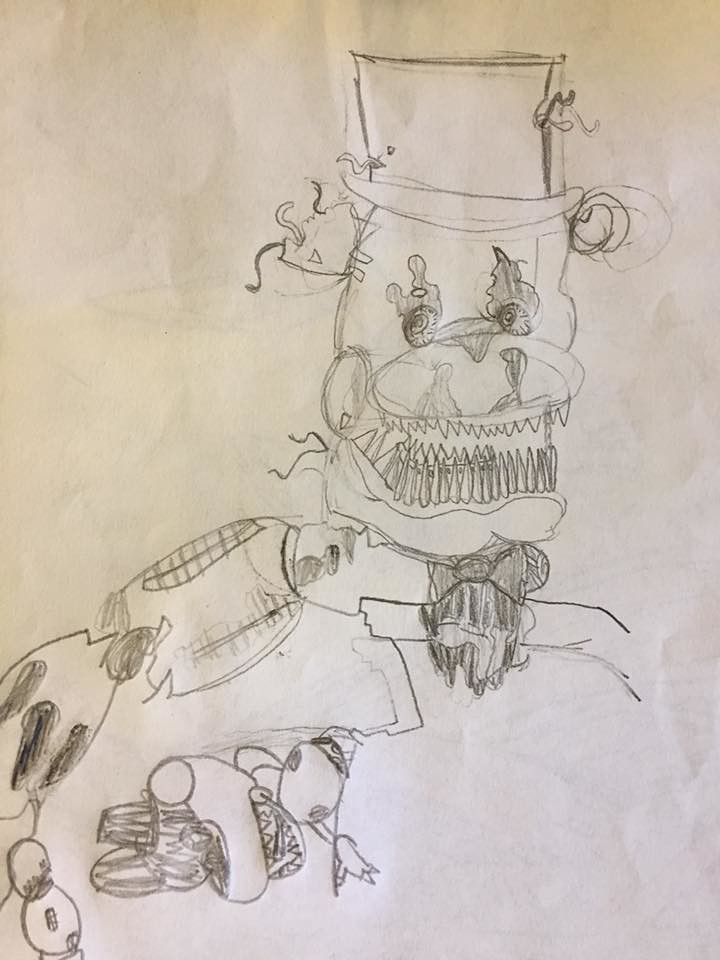In this detailed pencil drawing on a white piece of paper, a menacing bear-like creature is depicted at the center. The bear wears a classic top hat and has intensely dark eyes encircled by flame-like patterns, adding a sinister aura to its gaze. The creature's mouth is filled with rows of sharp, nail-like teeth on both the top and bottom jaws, emphasizing its ferocity. It is dressed in an elaborate outfit complete with a bow tie and a jacket. Notably, there is a small robot-like figure lying in the bottom left corner of the image. Additionally, the creature's shoulder features a mysterious device or item, adding to its mechanical and eerie appearance. This character bears a strong resemblance to those from the popular horror franchise, Five Nights at Freddy's.